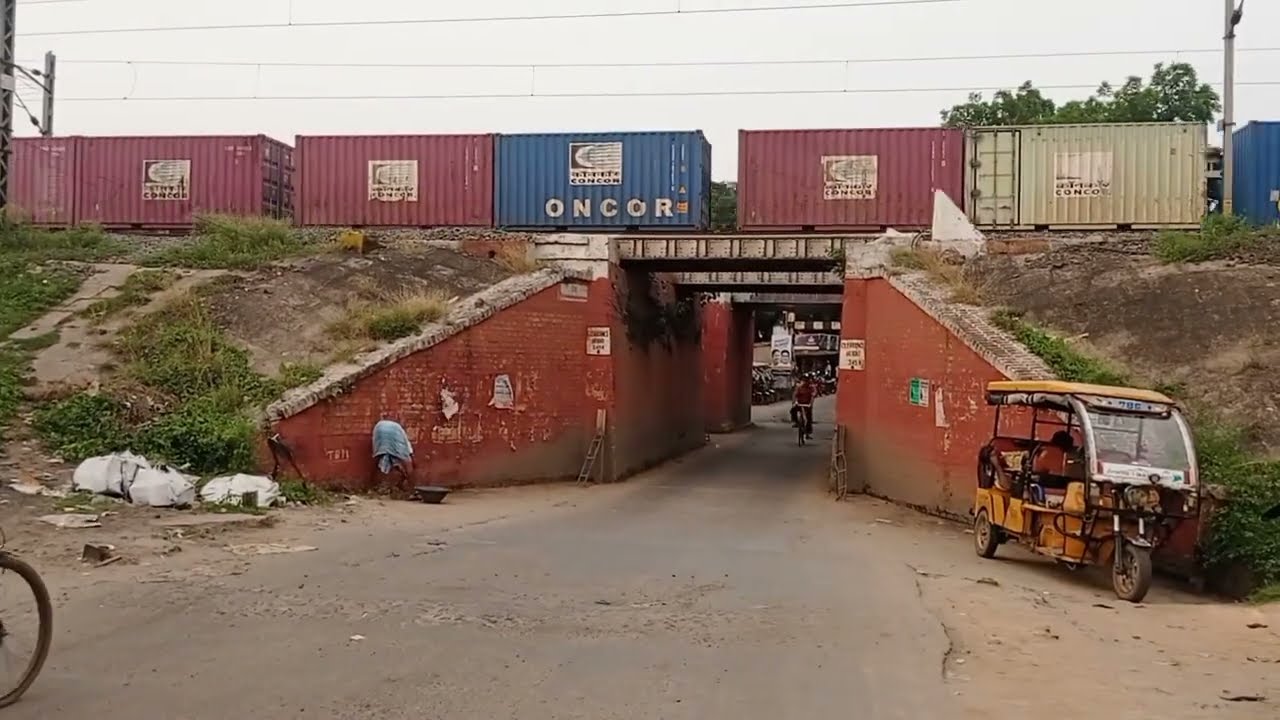This wide rectangular photo captures a bustling scene beneath a railway bridge, possibly situated in an Asian city like in India. The bridge itself supports a series of colorful cargo vans—grayish red, grayish blue, and light greenish gray—each adorned with a white square logo. Above the train track, telephone poles and wires can be seen extending across the top of the image. Beneath the tracks, a dark purple brick bridge with sloped grass and dirt patches on either side forms a tunnel. Emerging from this tunnel is a person in a red shirt riding a bicycle. To the right bottom portion of the image, there's a tri-cart with a plexiglass front and seating inside, possibly a food vendor or passenger vehicle, highlighting the city's vibrant street life. The scene is framed by reddish brick walls and bushes lining the slopes up to the train tracks, adding to the vivid and dynamic urban landscape depicted in this photo.